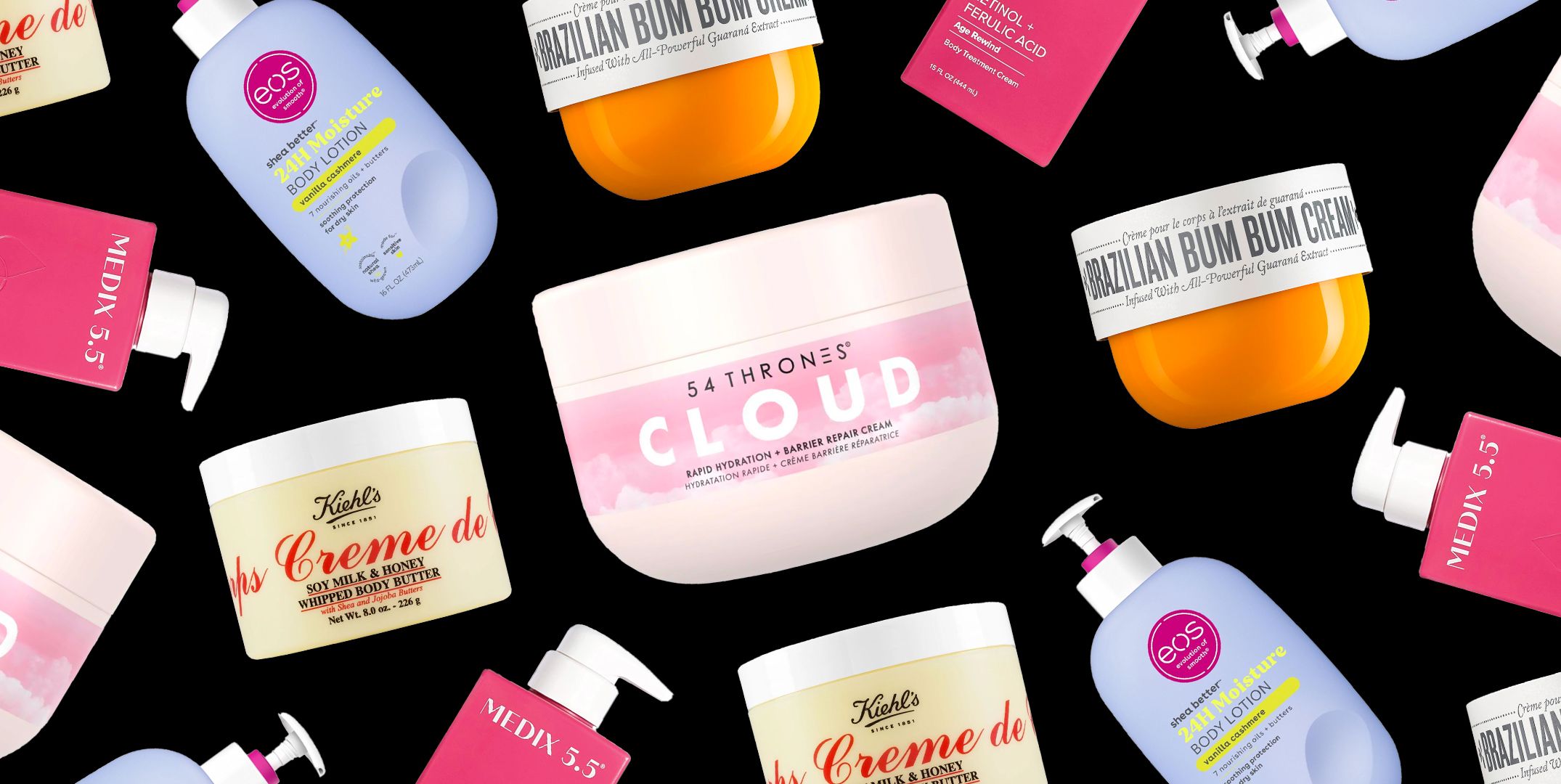This image showcases a diverse collection of health, wellness, and beauty products displayed against a black background. It includes predominantly pink, orange, and teal-containered items, with each product distinct yet complementary in its colorful presentation.

At the center of the image is a white container labeled "Cloud," part of the "54 Thrones" line, boasting "Rapid Hydration and Barrier Repair Cream." Surrounding it are other notable products like the "Brazilian Bum Bum Cream" in its recognizable orange container with a white top, and the "Kiehl's Soy Milk and Honey Whipped Body Butter," which comes in a cream-colored package.

Visible as well are several pink cylindrical containers marked "Medix 5.5," which appear to have pump tops, adding variation to the array. Alongside these is the "EOS 24 Hours Moisture Body Lotion," presented in a teal-colored container.

The arrangement of these 16 different products, including the repetitions of some, seamlessly blends various hues and shapes into a cohesive display of modern beauty essentials.